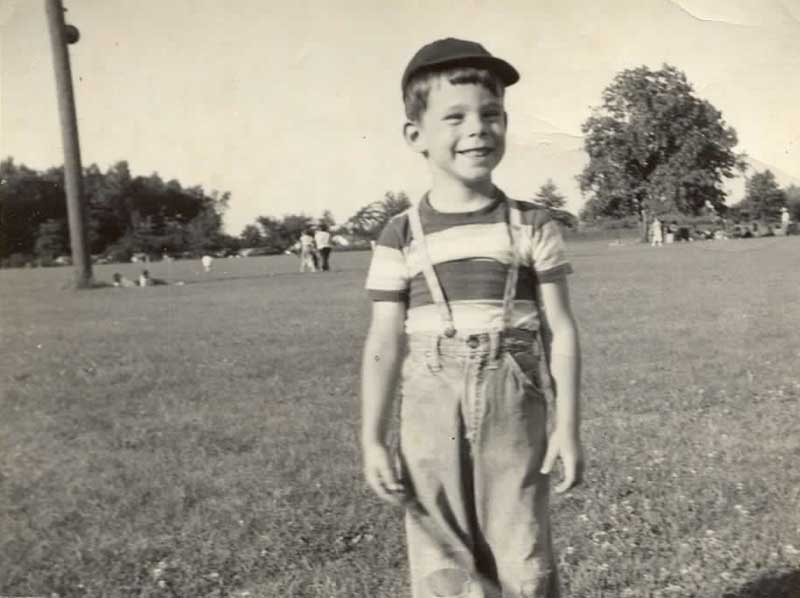This is a scanned black-and-white photograph likely from the 1930s, 40s, or 50s, depicting a cheerful young boy standing in a vast grassy field. The boy, who appears to be around six years old, is dressed in denim overalls with suspenders over a striped shirt. He wears a dark baseball cap and sports short, unevenly cut hair. His wide, joyful smile radiates happiness. In the background, several individuals are scattered across the field, either lounging or walking, enjoying what seems to be a pleasant summer day. Various trees and a light pole dot the field, with a gathering of people noticeable to the far right, adding to the lively outdoor scene.